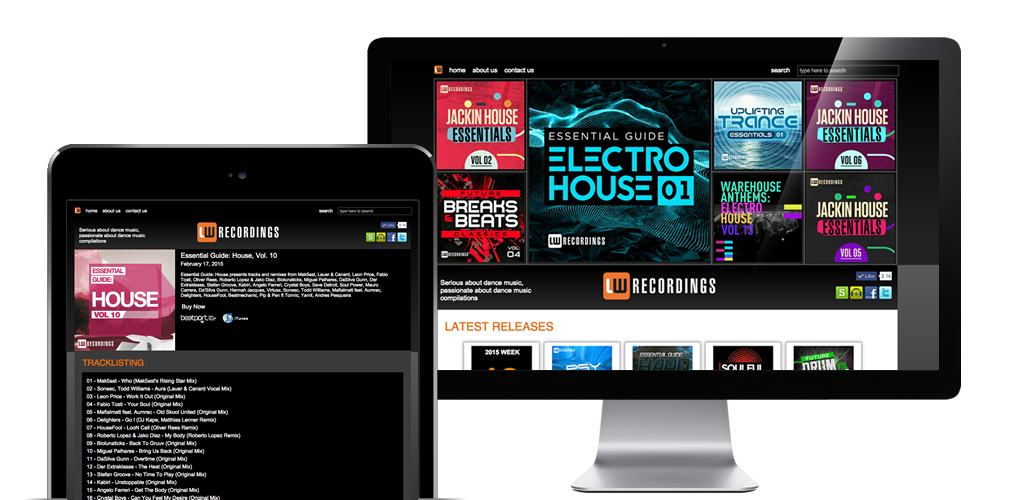In this image, there are two electronic devices showcasing the LW Recordings website. On the left is an Apple iPad, partially cropped, displaying the front view where the active screen reveals a black-themed webpage. The iPad, encased in black, features a discernible portion of the webpage, which seamlessly blends with the device's bezel. To the right is an iMac monitor, characterized by its black bezel and a sleek, silver, center-mounted metal base. The iMac exhibits a different section of the LW Recordings website, displaying album thumbnails against a white or transparent background, offering a contrast to the iPad’s display. The composition of the image highlights the visual consistency of the LW Recordings website across different Apple devices.